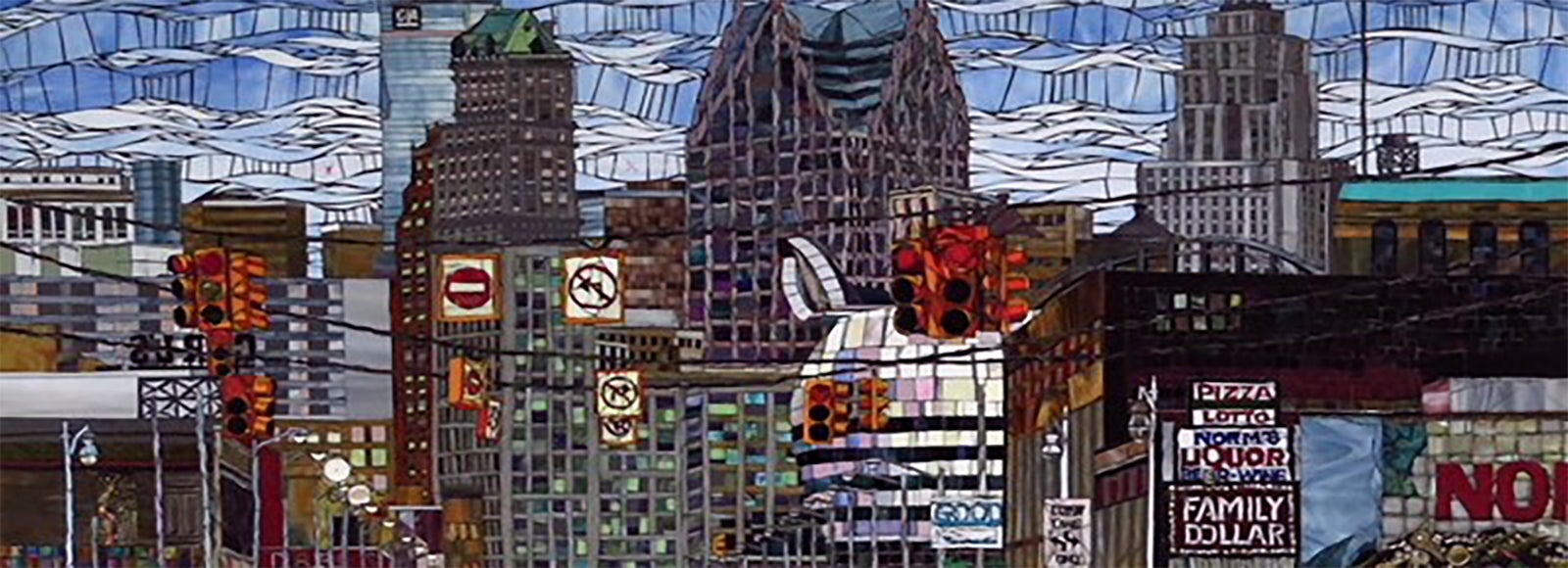This vibrant piece of art, possibly a mosaic or a painting with a mosaic-like style, depicts an urban cityscape dominated by towering skyscrapers and smaller buildings. The upper third of the image is filled with a sky composed of blue hues interspersed with white, resembling a stained glass or cubist design that could represent clouds or possibly water. Amidst the skyline, three primary skyscrapers stand prominent, with a variety of smaller structures filling the lower two-thirds of the composition.

In the foreground, a series of street signs and traffic lights are intricately depicted, hanging from black wires strung across the scene. These signs include Do Not Enter, No Left Turn, No Right Turn, and Wrong Way, adding to the bustling city vibe. Several commercial signs on the buildings read "Family Dollar," "Norm's Liquor," "Pizza," and "Lotto," while a partially visible "N-O" in red on a brick wall suggests other more fragmented advertising.

The buildings are depicted in muted tones of browns, grays, and blacks with black-outlined windows, enhancing the urban atmosphere. Street lamps dot the scene, adding to the depth and realism of the streetscape. The careful arrangement and layering of the tiles or paint create a richly detailed and dynamic representation of a downtown area, blending elements of cubism and mosaic art to vividly capture the essence of city life.